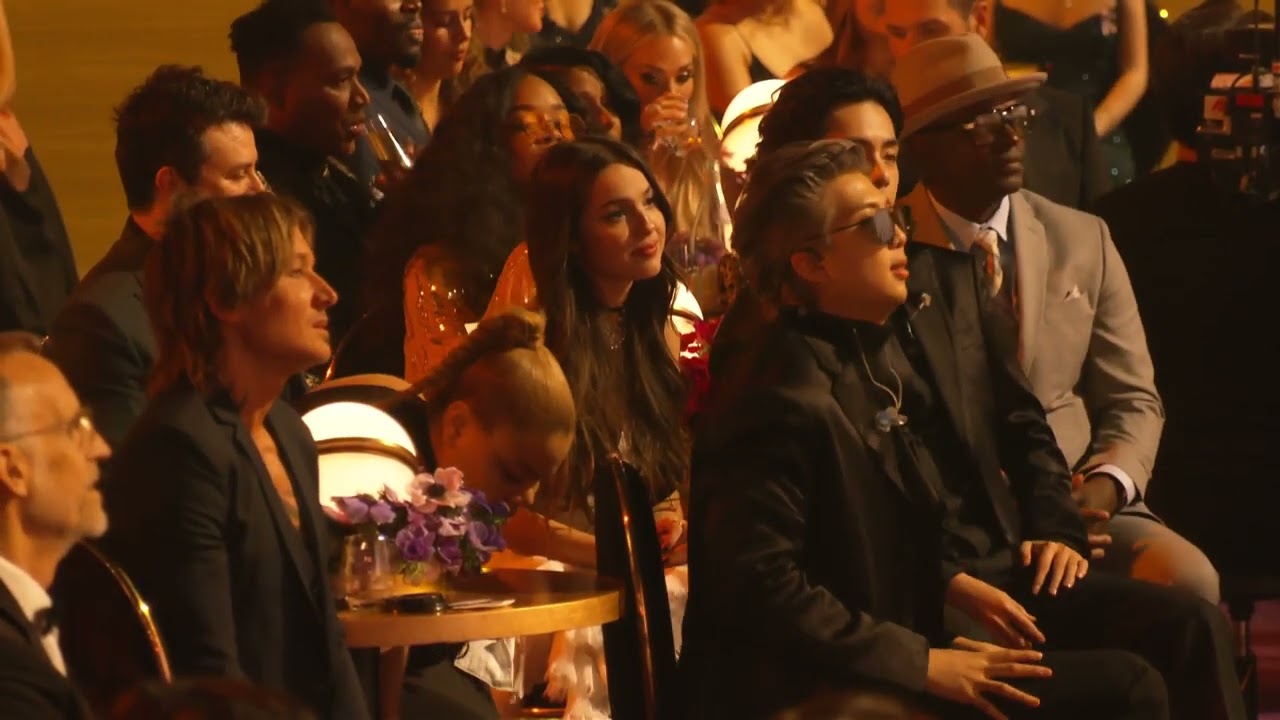This image appears to be from a prestigious event, likely the Country Music Awards, featuring a diverse crowd intently watching a stage to the right. In the foreground, country music star Keith Urban is easily recognizable. Beside him, possibly with red hair in a high ponytail, sits a woman who might be his wife, Nicole Kidman. The attendees, representing various nationalities, include an Asian man in a black tux and dark glasses, and an African-American man in the front row wearing glasses, a tan suit jacket, a tie, and a country-western hat. Amidst the crowd, which is seated and enjoying drinks, a woman who resembles Queen Latifah is bending down near a small table adorned with flowers and what might be a small globe light. Everyone's attention is captured by the unseen spectacle on stage.